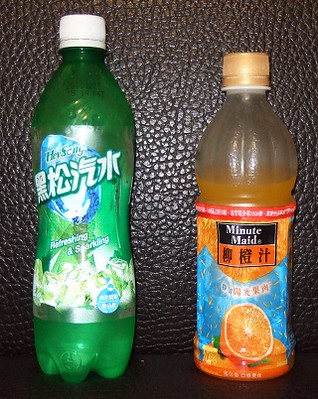The photograph features a textured background that resembles dark, blackish-brown leather, characterized by its bumpy surface, with lighter high points giving it a tactile appearance. At the bottom of the photograph, there is a smooth, black tabletop. Positioned prominently on the tabletop are two beverage bottles. 

On the left, there is a green plastic bottle that appears to be a soda, potentially Sprite. It has a distinctive curvy shape at its round base and is sealed with a white cap. The bottle's label showcases Asian characters, suggesting it is an international variant of the drink.

Next to it, on the right, is a smaller bottle of Minute Maid orange juice. This bottle also has a white cap and features a label adorned with Asian characters, indicating its international origin. Notably, the bottle of orange juice is partially consumed, with the liquid level visibly lower inside the transparent container.